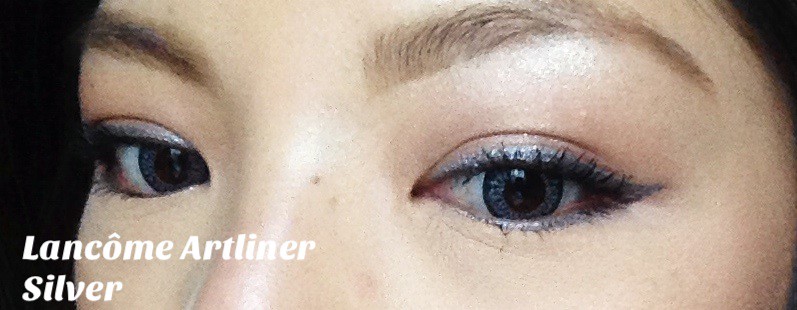This is an extremely detailed, close-up image focusing on a woman’s eyes, likely of Asian descent, with only her eye region visible. Her complexion appears pale, and her eyes—a striking bright blue, suggesting she may be wearing contacts—look slightly downward. Her light brown eyebrows are well-defined, shaping her expression. The eye makeup she's wearing is a glittery light blue, applied in a cat-eye style, complemented by thick black mascara. A hint of her dark hair is visible in the top right corner of the image, while the background on the left edge is black, possibly her hair or the backdrop. In the bottom left corner of the image, the text "Lancôme Art Liner Silver" is boldly italicized in white, indicating the purpose of the image might be to showcase this specific eyeliner product.